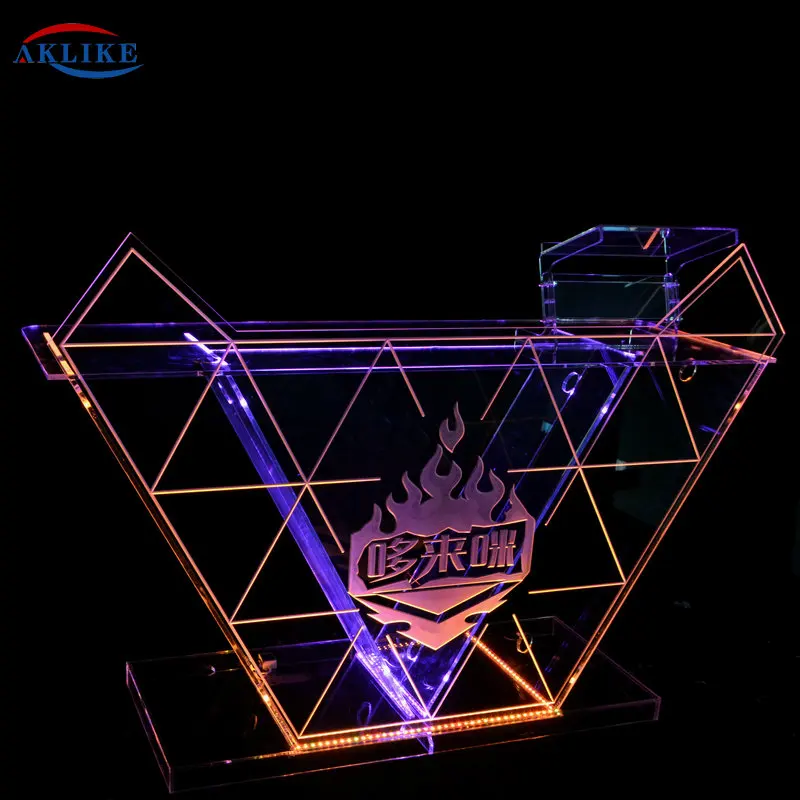The image depicts an elaborate, futuristic frame that could easily be a feature in a Japanese TV show obstacle course. The structure is distinctly geometric, primarily formed of rhombuses, triangles, and trapezoids, and is illuminated with vivid neon tubing. The main sections radiate an orangish glow, accentuated by occasional stripes of bluish-purple light. Dominating the center is an emblem adorned with flames, inscribed with characters that appear to be in Japanese or Chinese. The precise meaning of the text remains unclear. In the upper left-hand corner, the acronym "A-K-L-I-K-E" is prominently displayed in block letters, encircled by a red arc above and a blue arc below. The entire figure has a complex, metallic and glass structure with see-through plastic elements, emphasizing its futuristic and high-tech aesthetic.